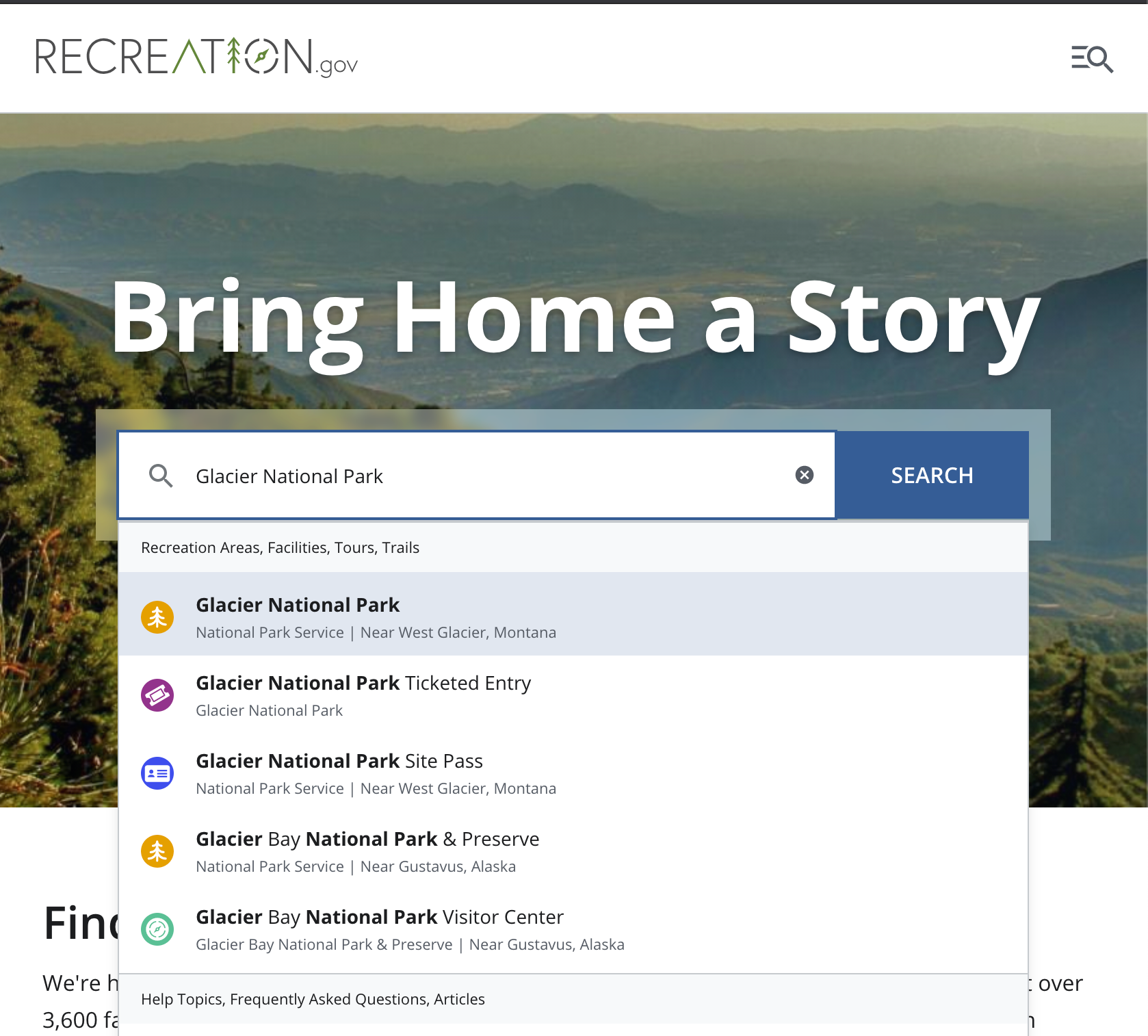This image, sourced from recreation.gov, features a structured layout with distinct elements. At the top of the image is a thin black line extending horizontally from the left to the right edge. Immediately beneath this line, a white bar displays the text "RECREATION.gov." The text "RECREATION" appears in all capital letters with a black font, while ".gov" is rendered in a smaller font size. Notably, the letter "A" in "RECREATION" is stylized as the top part of a triangle, the "I" is designed to resemble a tree symbol, and the "O" has a unique design that gives it an appearance reminiscent of a whale's eye.

Below the white bar, the image transitions into a photograph of a scenic outdoor landscape that resembles a canyon. The photograph showcases a mix of rugged mountains and hilltops flanking a central area of flat land, capturing the essence of the canyon environment. Overlaying this picturesque scene is white text that reads, "Bring Home a Story."

At the bottom center of the image, a search bar prominently displays the text "Glacier National Park." A dropdown menu beneath the search bar lists five results related to Glacier National Park, suggesting possible destinations or articles connected to the search query. This comprehensive and visually appealing image effectively combines branding elements with an invitation to explore natural wonders.